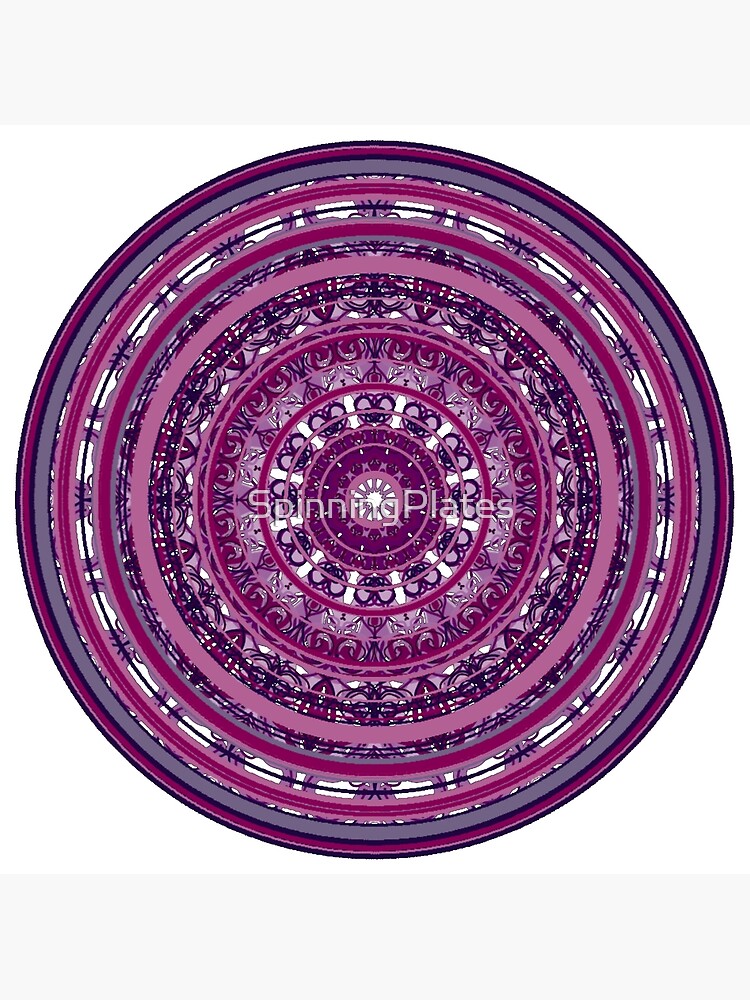The image depicts a detailed purple circular design composed of concentric rings with intricate flowery and geometric patterns. These patterns, rendered in various shades of purple ranging from dark to light, create a visually complex and ornate effect that resembles a decorative plate or rug. The outermost ring is dark purple, followed by subsequent rings in gray and lighter shades of purple, interspersed with floral designs, crowns, and miscellaneous geometric shapes. The central area features a motif resembling a ship's wheel. Superimposed over the middle of the design is a watermark with the text "Spinning Plates" in light gray or white, partially obscured by the intricate background. The entire composition is set against a solid white backdrop, enhancing the vividness and detail of the purple concentric patterns.